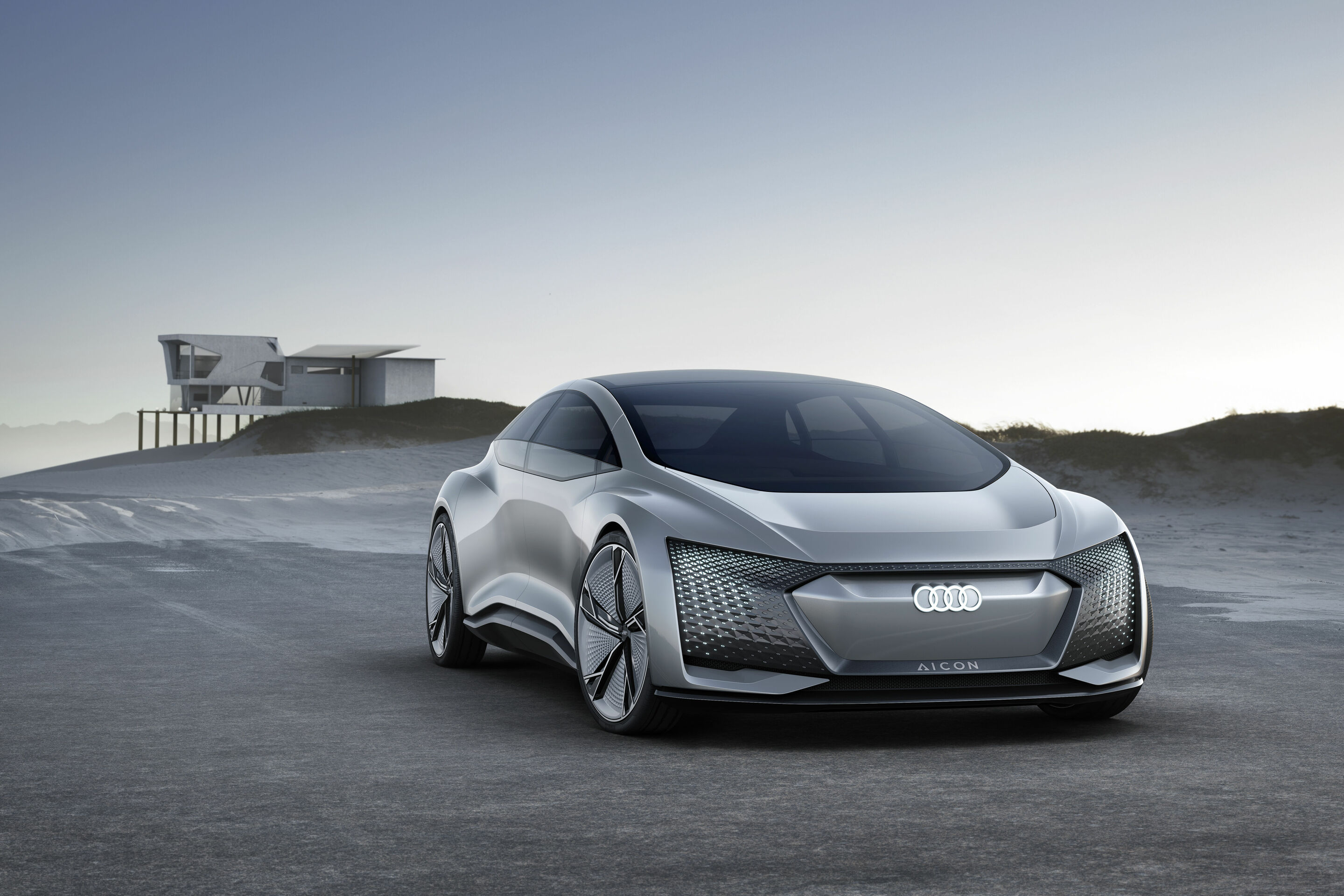The image showcases a computer-simulated, highly futuristic Audi vehicle, prominently featuring the iconic Audi four-ring emblem on the front. The car, labeled with "AI CON” on what appears to be its number plate, epitomizes sleek modernity through its streamlined design. Its overall shape hints at Audi's classic coupe models while introducing entirely new, unprecedented elements. The vehicle resembles a high-tech prototype or artistic sketch of an avant-garde electric car. Its contemporary aesthetic includes substantial, futuristic wheels with a slight Tesla resemblance, an expansive, window-heavy roof, and a unique black grill structure, all enveloped in a sleek grey finish. There are no visible door handles, enhancing its minimalist design. The background includes a distant house, likely on a platform extending over water, with what seems to be a beach to the image's right and a mountainous horizon. The car is depicted on a stretch of grey road with patches of grass to the side, in what appears to be a black and white scene.